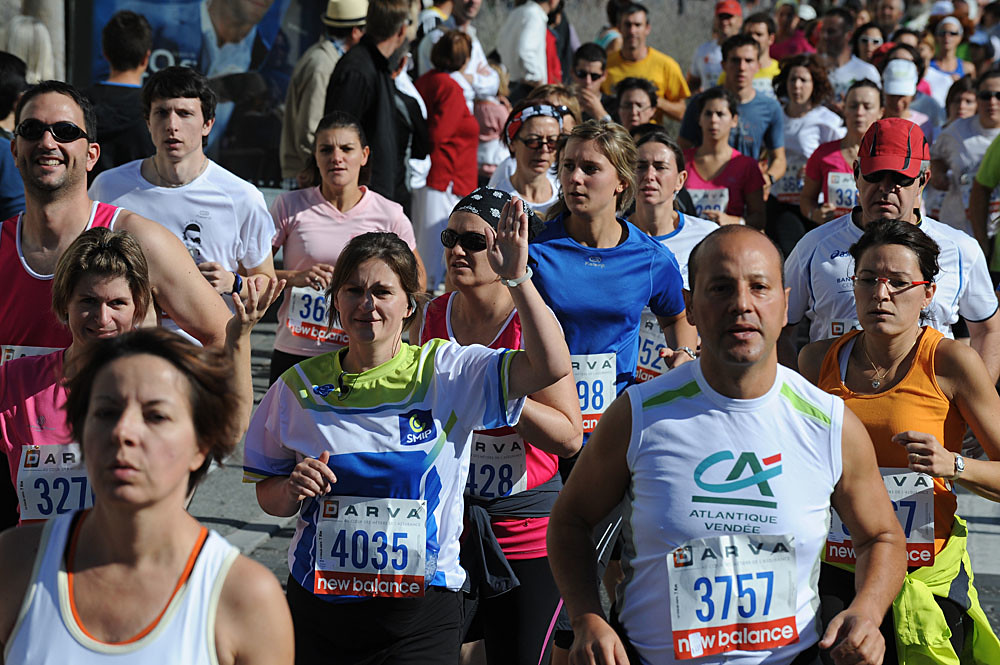In this outdoor daytime photograph capturing the energy and motion of a marathon, a large, diverse group of at least fifty to sixty runners is depicted participating in a race. The runners, primarily wearing tank tops and short-sleeve shirts, are adorned with numbered bibs prominently displaying the New Balance brand. Key figures in the foreground include a man in a white tank top with the text "Atlantique Vendee" and bib number 3757, accompanied by a woman in a white t-shirt marked with "SMP" and bib number 4035. Another notable participant is a woman in a white tank top whose bib is obscured. Surrounding them are runners in various colored attire: a woman in red with bib number 327, a man in a red tank top, a woman in a headscarf and red tank top, a young woman in a black t-shirt with a partly-obscured bib beginning with 98, a man in a red baseball cap, and a woman in an orange tank top. Among the sea of runners, some participants are seen smiling or waving at the camera, while the rest are focused on the race. The background is filled with additional runners and spectators observing the event, emphasizing the scale and enthusiasm of the occasion.